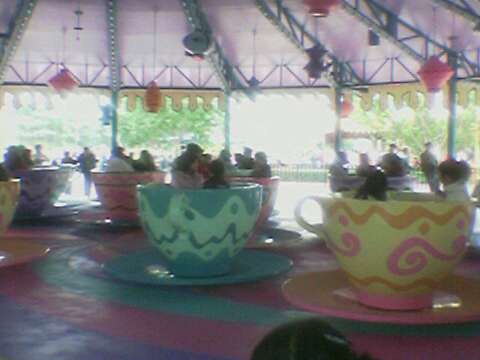The image captures the lively interior of a covered teacup ride, reminiscent of Disneyland, set within an amusement park or carnival. The ride is housed under a large purple canopy adorned with yellow drippings, creating a whimsical atmosphere. In the foreground, a somewhat blurred green teacup sits on a matching green saucer, featuring a dark green scallop design along the top and bottom, with a lighter green in the middle. Nearby, a yellow teacup with an orange zigzag pattern and pink swirl designs stands out. Additional teacups in varying colors, such as blue with green patterns, spin around in the background. The scene is animated with men, women, and children either seated inside the teacups or standing around, adding to the dynamic motion captured in the photograph. Above the ride, oriental lanterns of different designs hang from the rafters, alongside speakers and various lighting fixtures, while sunlight and greenery peek through from the ride’s perimeter.